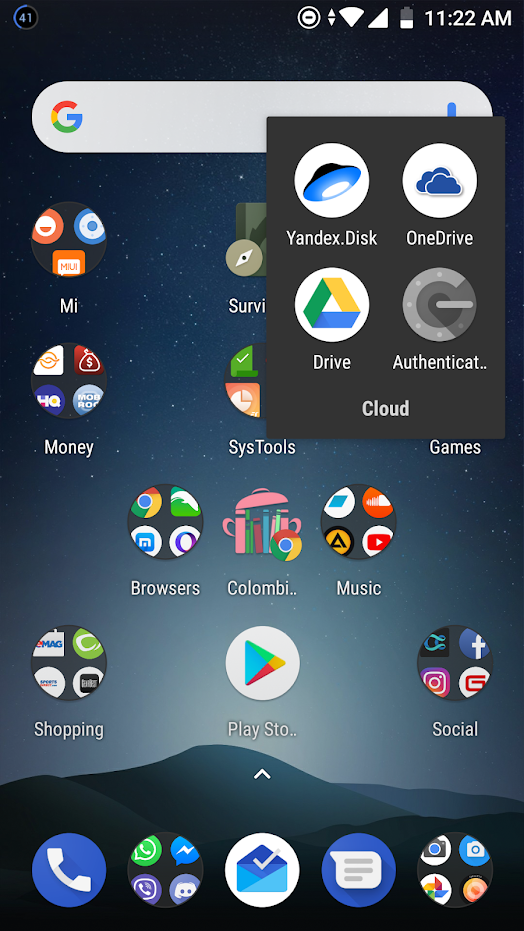In this image, we see the home screen of an Android device. In the top-left corner, the battery percentage is displayed at 41%. To the right, the status bar shows the 'Do Not Disturb' icon, the Wi-Fi connection icon, and the network signal bar with full strength. Additionally, the battery level indicator is visible, and the time is shown as 11:22 AM.

The home screen includes various apps such as Yandex.Disk, OneDrive, Drive, Authenticator, and Mi Folder. There are also categorized folders for Money, Sister, Browsers, and Music. Commonly used apps like the dialer, messaging, email, camera, photos, WhatsApp Messenger, and Discord are also present.

The background image of the home screen features a serene blue hue with a mountain landscape at the bottom.